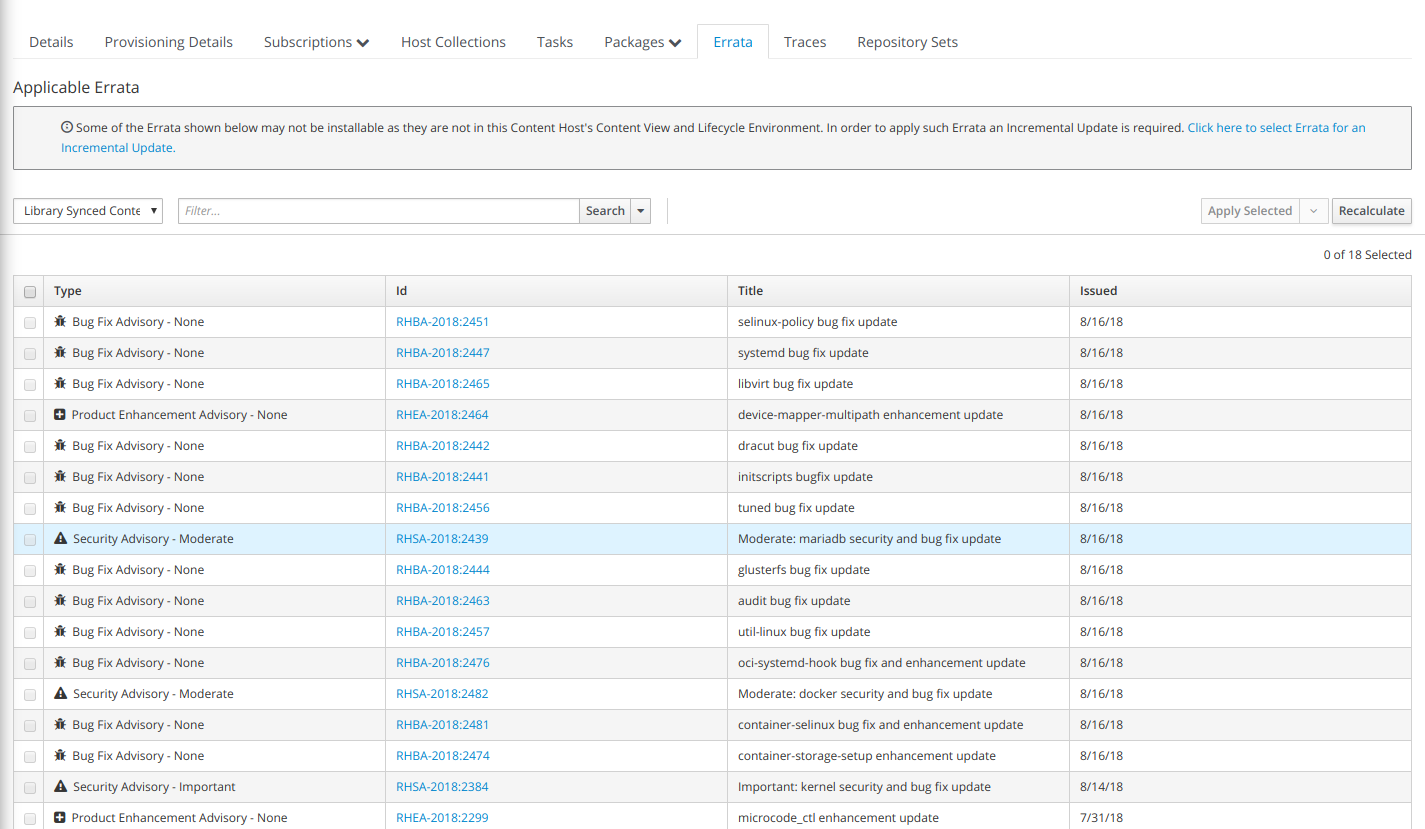A screenshot of a webpage detailing various system management and maintenance tasks is depicted. At the very top, from left to right, the header features several tabs labeled "Details," "Provision Details," "Collections," "Tasks," "Packages," "Errata," "Traces," and "Repository Sets." Due to the small font size, these labels are not easily readable.

Below the header, the section titled "Applicable Errata" is displayed. Following this, there is a subsection labeled "Library Synced Content," which lists various items in a systematic format. The items are categorized under several headers including "Type," "ID," and "Title." The "Type" column includes categories such as "Bug Fix Advisory," "Product Enhancement Advisory," and "Security Advisory."

Each row under these headers includes an ID number and a brief description of the content. For instance, typical entries in this list might include titles like "Bug Fix Update," "System Bug Fix Update," and "Security Advisory," with corresponding descriptions mentioning specifics such as "Incorporate Kernel Security." There are an estimated 20 items displayed in this organized table, each one specifying issues related to system bugs, advisories, and security updates, likely intended for reviewing and managing updates on computer or mobile devices.